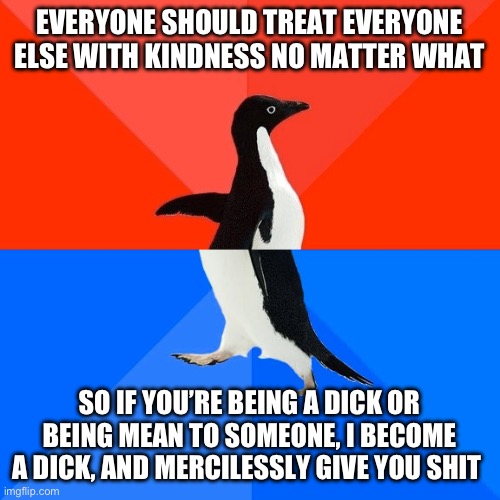This meme employs a well-known format featuring a penguin. The image is divided into two halves: the upper portion has a red background, while the lower portion is blue. In the top half, the penguin is shown moving in one direction, accompanied by text that reads: "Everyone should treat everyone else with kindness no matter what." In the bottom half, the penguin appears to be moving in the opposite direction, paired with text that says: "So if you're being a dick or being mean to someone, I become a dick and mercilessly give you shit." This meme highlights the duality and conditionality often found in social interactions, emphasizing the idea of treating others the way they treat you.